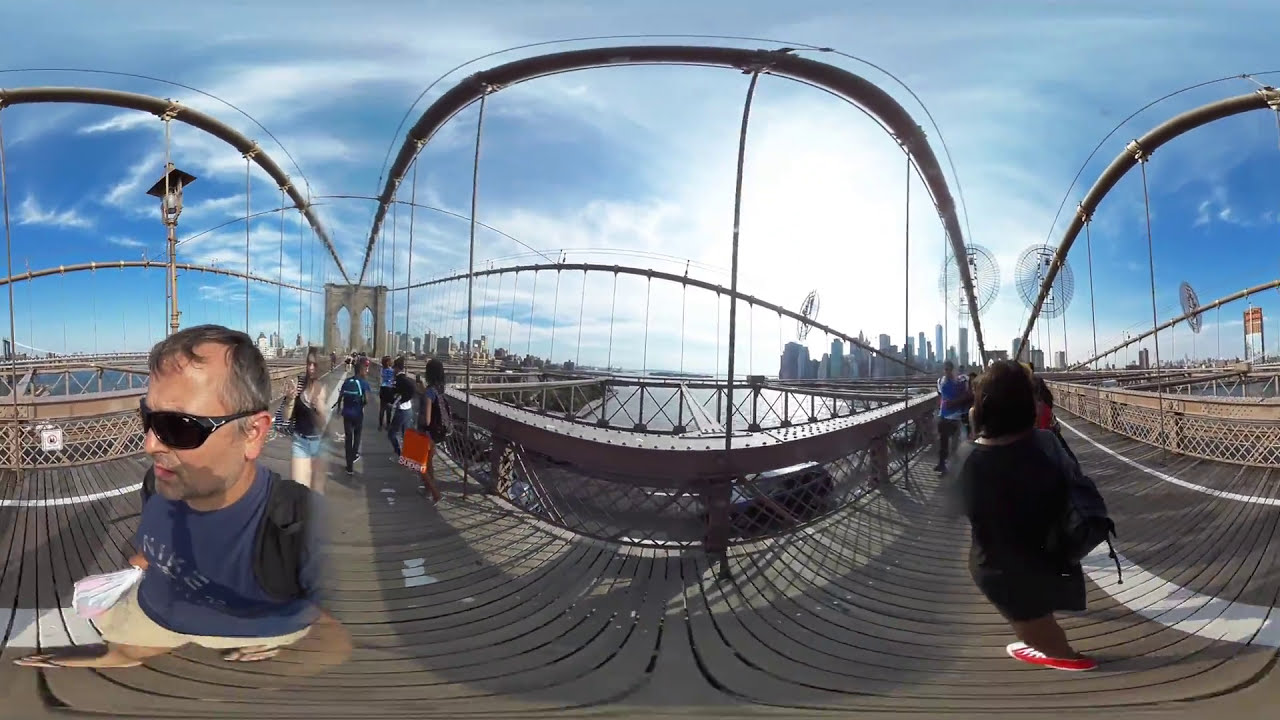A distorted image of the iconic Brooklyn Bridge captures a surreal scene where New York City appears at both ends of the bridge, seemingly bending at the center. The bridge's cement columns and cables are prominently visible, although the distortion makes the paths of three cables unclear. The photograph showcases the large arches and suspender cables that span the structure, all set against a bright blue sky dotted with a few wispy clouds, indicating a sunny summer day. 

In the foreground to the left, a middle-aged man with short, salt-and-pepper hair is walking along the wooden planks, wearing sunglasses, a blue Nike t-shirt, beige shorts, and flip-flops. He is also carrying a white bag and sporting a black backpack. On the right side, a woman, dressed entirely in black with red Converse tennis shoes, walks in the opposite direction, her back turned to the camera. Additional pedestrians are visible scattered across the bridge, contributing to the lively atmosphere. The river below the bridge glimmers under the sunlight, completing the scenic urban tableau with distant skyscrapers framing the scene from both sides.